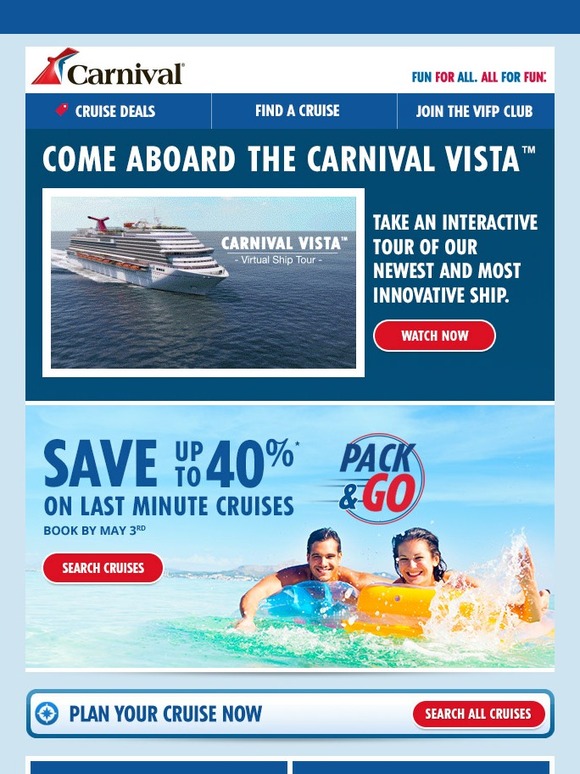This is a screenshot of a vibrant and enticing Carnival Cruise advertisement. At the very top, there's a thin blue bar. Below this, the iconic Carnival logo is prominently displayed, resembling a red airplane wing or fin. On the right-hand side of the logo, the catchy slogan "FUN FOR ALL. ALL FOR FUN." is written in alternating blue and magenta letters. The menu offers three distinct options: "Cruise Deals," "Find a Cruise," and "Join the VIFP Club."

Dominating the center of the ad is a large blue rectangle featuring bold, white, all-capitalized text that invites viewers to "COME ABOARD THE CARNIVAL VISTA." Accompanying this text is a stunning image of a Carnival cruise ship cutting through the water, framed by a white border. Below the image, a promotional phrase reads, "Take an interactive tour of our newest and most innovative ship," followed by a red button urging viewers to "WATCH NOW."

Further down, another advertisement features a playful scene of two individuals enjoying the water on inflatable pool toys. A man floats on a blue toy while a woman relaxes on a yellow one. The image is accompanied by a compelling offer: "Save up to 40% on last-minute cruises booked by May 3rd." Next to this promotion, there is a "Search Cruises" option and a "Pack and Go" reminder.

At the very bottom of the screen, a long rectangular section appears. On the left side, the text "Plan Your Cruise Now" is displayed in blue, while the right side features a red button that encourages viewers to "Search All Cruises."